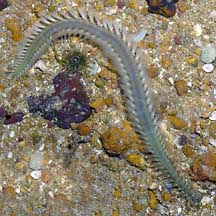The image depicts an underwater scene featuring a long, snake-like creature that appears to be a centipede or marine worm. This silvery gray organism is situated on a rocky, sandy bed and stretches from the bottom right corner to the top left of the picture. The creature has numerous leg-like structures along its narrow, tube-like body, and it twists as it moves. The underwater environment is filled with sparkling flakes of crystals and rocks in various colors, including clear, white, gray, gold, purple, green, orange, navy blue, dark reddish shades, and black. The water is clear, offering a view of the sandy, rocky terrain that forms the underwater bed. There's no text in the picture, just a rich palette of colors and the snake-like creature set against the aquatic backdrop.